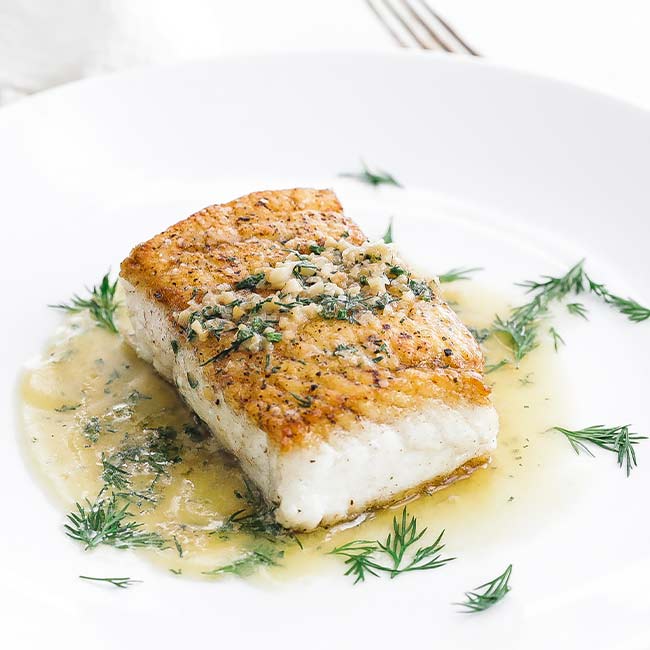The photograph showcases a close-up of a square-shaped, gourmet fish dish served on a pristine white plate. The plate features a distinctive design with a lower front and a gently sloped rim along its edge. It occupies approximately 80% of the image from top to bottom, revealing only a semi-circular portion at the top, while the left, right, and bottom edges remain outside the frame.

At the center of the plate lies a rectangular block of white fish, most likely a couple of inches in width, three to four inches in length, and around an inch in height, positioned at a slight angle. The fish’s surface is beautifully browned, providing a textured contrast to its otherwise white flesh. Adorning the top are small, finely chopped pieces of garlic, arranged in a neat strip along with an abundance of finely chopped herbs, possibly chervil, given their small, pointed leaf structure.

Beneath the fish, a luxurious buttery sauce is artfully spread in an irregular shape, with darker hues on the left side and lighter on the right, adding a rich and creamy base to the dish. The meticulous presentation and the harmonious blend of colors and textures elevate this simple fish dish into a visually appealing culinary masterpiece.